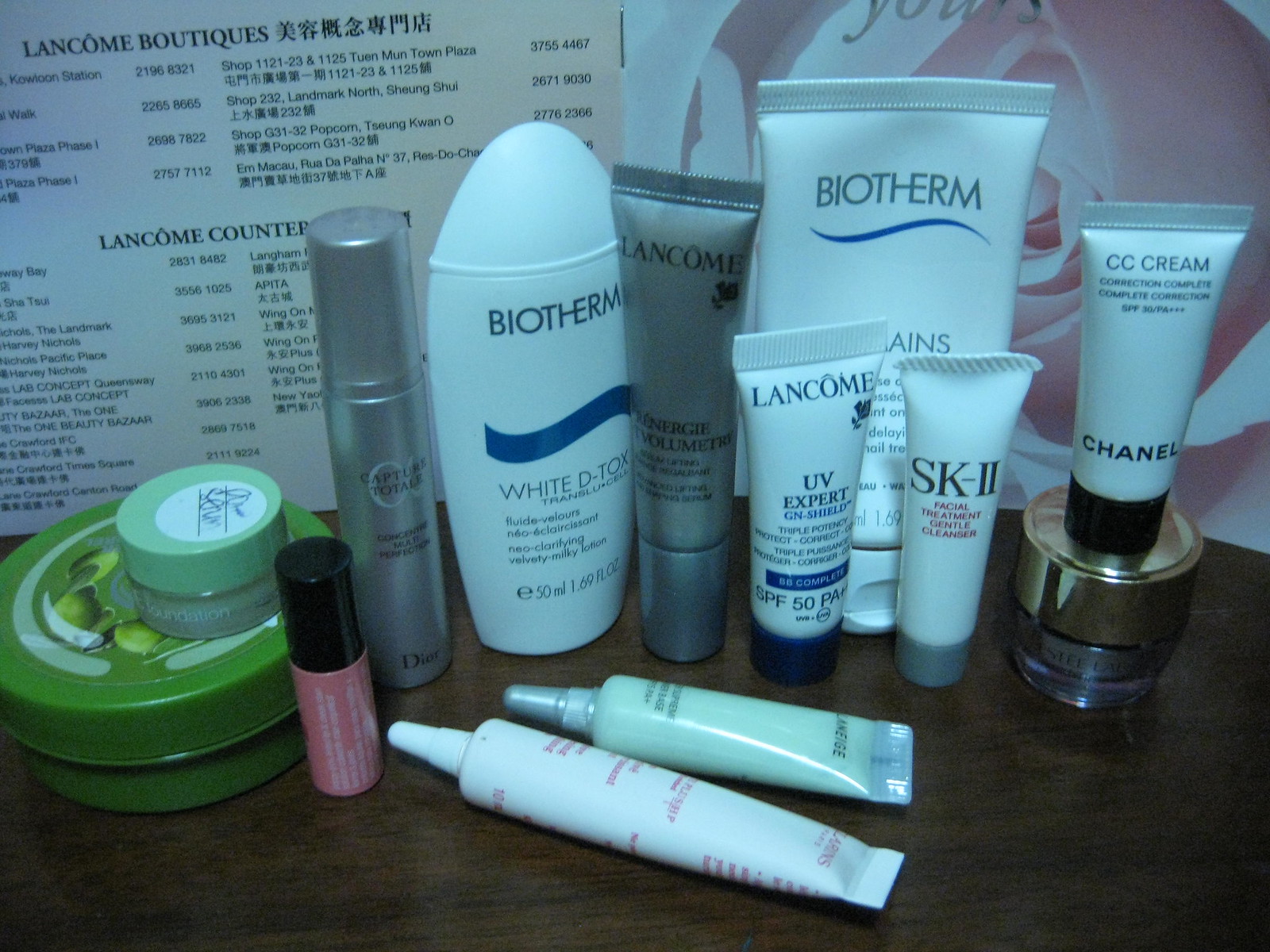The image captures a neatly arranged collection of beauty products displayed on a countertop, likely in a bathroom or a dresser area. The countertop itself features a rich, dark brown wood grain finish with what seems to be rounded edges, although the exact meeting point with the wall isn't visible.

From left to right, the arrangement begins with a large green jar that has a floral-themed label, suggesting a botanical or organic product. Stacked on top of this jar is a smaller, mint green jar, adding a touch of pastel color to the setup. To the right of these jars is a small pink tube with a black cap, possibly containing lip gloss. 

Next in line is a cylindrical gray tube labeled "Capture Total from Dior," exuding a sense of luxury. Following this is a bottle labeled "Biotherm White Detox," indicating a skincare product focused on whitening or clarifying the skin. Another gray tube comes next, labeled "Lancôme Volumetri," suggesting a volumizing treatment, perhaps for eyes or face. 

Adjacent to this is a bottle of "Lancôme UV Expert Shield," a product likely intended for sun protection. Following this, there's an "SK-II Facial Treatment Gentle Cleanser," representing a high-end facial cleanser. Next is an "ACC Cream" from Chanel, denoting another high-end skincare item. 

Finally, the arrangement concludes with another jar at the far right, alongside two smaller, unlabeled tubes positioned in front of the main lineup. The exact details of these smaller tubes are unclear, but they add to the overall sense of a well-curated and comprehensive beauty regimen.